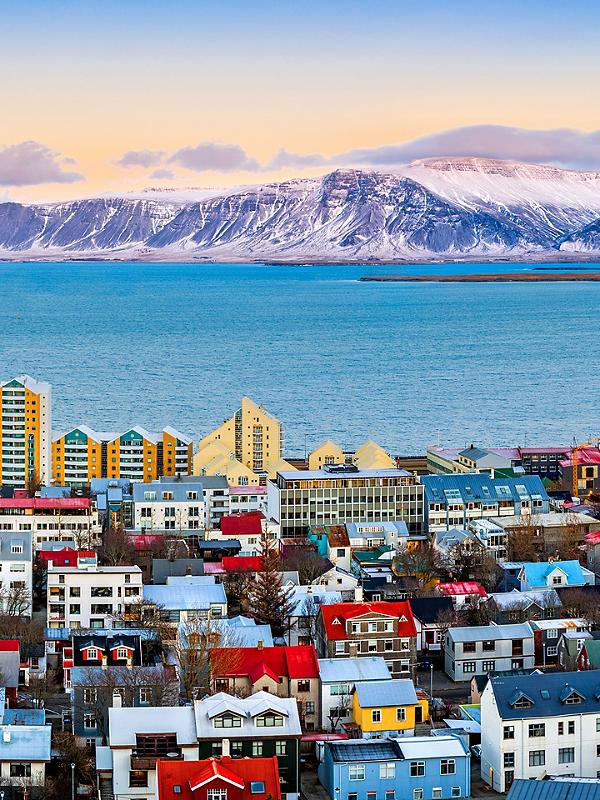The image depicts a vibrant arctic city nestled near a large, serene body of blue water. The town consists of numerous 1 to 3-story houses, painted in a spectrum of bright colors—red, blue, white—and some adorned with red roofs. Treetops and small pine trees intersperse the buildings, giving the scene a cozy, tightly packed feel. Towards the water's edge, larger buildings, resembling condos and varying from 5 to 10 stories, stand prominently. In the background, an imposing glacier or mountain, intricately marked with snow and icy blue crevices, stretches towards a sky colored in hues of light blue and pinkish-orange, streaked with gray puffy clouds. This picturesque arctic landscape, possibly painted during the tranquil moments of sunset or sunrise, captures the beauty and unique structure of this northern city.